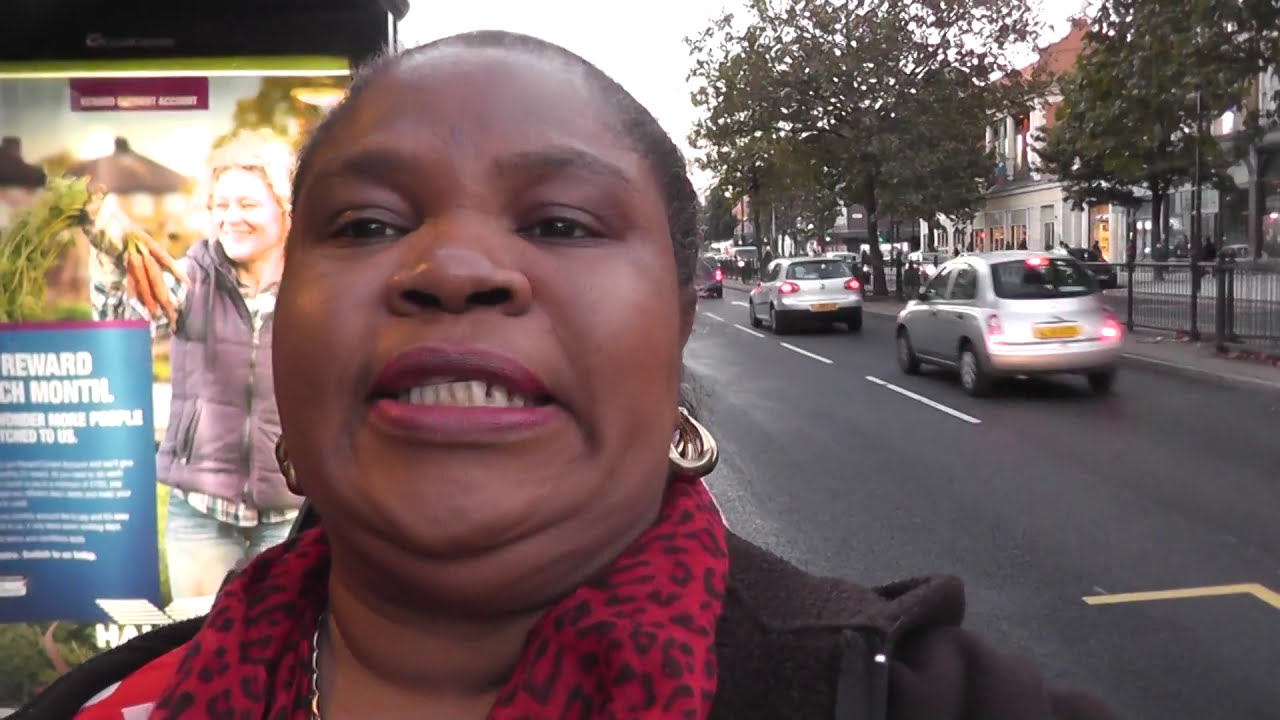The photograph captures a dark-skinned woman with very short brown hair, dark eyes, and reddish lipstick, standing near the curb of a town roadway. She is wearing gold hoop earrings, a black jacket, and a red and black patterned scarf. Her mouth is partially open in an awkward grimace, revealing her teeth, while her head is tilted back slightly, causing a slight neck roll.

In the background, on the left-hand side of the image, there is a prominent advertisement sign with a black top frame and a green line below it, featuring an image of a blonde woman holding a bunch of carrots, set against a sky backdrop and a gazebo. The sign has text on a burgundy background, with partially readable words "reward" and "Montil" in white on a blue strip below a burgundy top strip, accompanied by some green grass and bushes.

On the right-hand side of the image, a blacktop road with dashed white lines and several silver cars (and one black car) moving away can be seen. The cars' brake lights are visible, indicating a waiting line, next to which lies a gray cement sidewalk with planted trees, boasting green leaves. The setting features buildings, including a white one with a red rooftop closer to the front and a distant brown building. A silver gate and pedestrians on the sidewalk add to the town's bustling atmosphere, captured under a white sky.